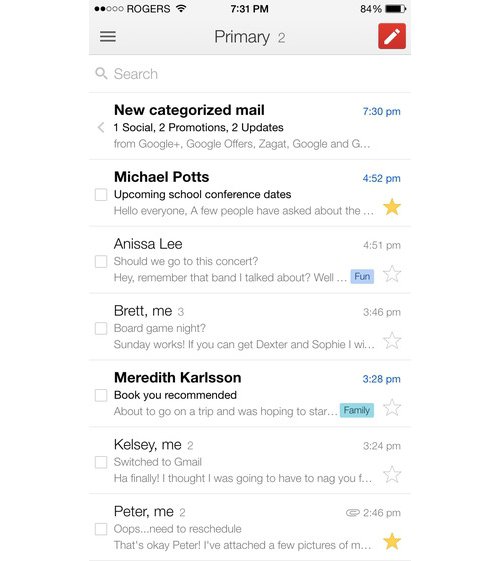The image appears to be a screenshot of either an email inbox or a search results list viewed on a smartphone or web interface. The interface is divided into several sections:

- **Top Section:** 
  - The title "Primary" is displayed prominently in black letters, followed by a smaller gray number "2". This is set against a gray background.
  - On the right-hand side, there is a red icon featuring a 45-degree angled pencil.

- **Search Bar:**
  - Directly below this is a white background containing a search bar on the left side.

- **Email/List Content:**
  - There are seven rows, each containing different pieces of information along with timestamps on the far right.

  1. **First Row:**
     - Title: "New categorized mail" in black.
     - Subcategories: "1 Social," "2 Promotions," and "2 Updates" all in smaller black letters.
     - Source information in light gray: "From Google Plus, Google Offers, Zagat..."
     - Timestamp: "7:30 PM" in blue letters.

  2. **Second Row:**
     - Sender: "Michael Potts" in dark black.
     - Subject: "Upcoming school conference dates" in gray.
     - Message Preview: "Hello, everyone. A few people have asked about the..." truncated with a yellow star to the right.
     - Timestamp: "4:52 PM" in blue letters.

  3. **Third Row:**
     - Sender: "Anissa Lee" in gray.
     - Subject: "Should we go to the concert?" in gray.
     - Message Preview: "Hey, remember that band I talked about? What..." truncated. There is a light blue square with a blank white star on the right.
     - Timestamp: "4:51 PM" in gray letters.

  4. **Fourth Row:**
     - Sender: "Brett, Me" with the number "3."
     - Subject: "Board game night?" in gray.
     - Message Preview: "Sunday works. If you can get Dexter and Sophie, IWI..." truncated with a blank white star.
     - Timestamp: Not explicitly mentioned.

  5. **Fifth Row:**
     - Sender: "Meredith Carlson" in dark black.
     - Subject: "Book you recommended" in black.
     - Message Preview: "About to go on a trip and was hoping to star..." truncated. Accompanying this is a teal blue rectangle that reads "Family" and a blank white star.
     - Timestamp: "3:28 PM" in blue letters.

  6. **Sixth Row:**
     - Sender: "Kelsey, Me" with the number "2" in gray.
     - Subject: "Switch to Gmail" in gray.
     - Message Preview: "Ha, finally! I thought I was going to have to nag you F..." truncated with a blank white star.
     - Timestamp: "3:24 PM" in gray letters.

  7. **Seventh Row:**
     - Sender: "Peter, Me" with the number "2" in gray.
     - Subject: "Oops..." in gray.
     - Message Preview: "Need to reschedule. That's okay, Peter. I've attached a few pictures of M..." truncated with a yellow star to the right.
     - Timestamp: "2:46 PM" in light gray letters.

This detailed description provides an organized view of an email or search list divided into distinct sections, showcasing various senders, subjects, and message previews, each with corresponding timestamps.